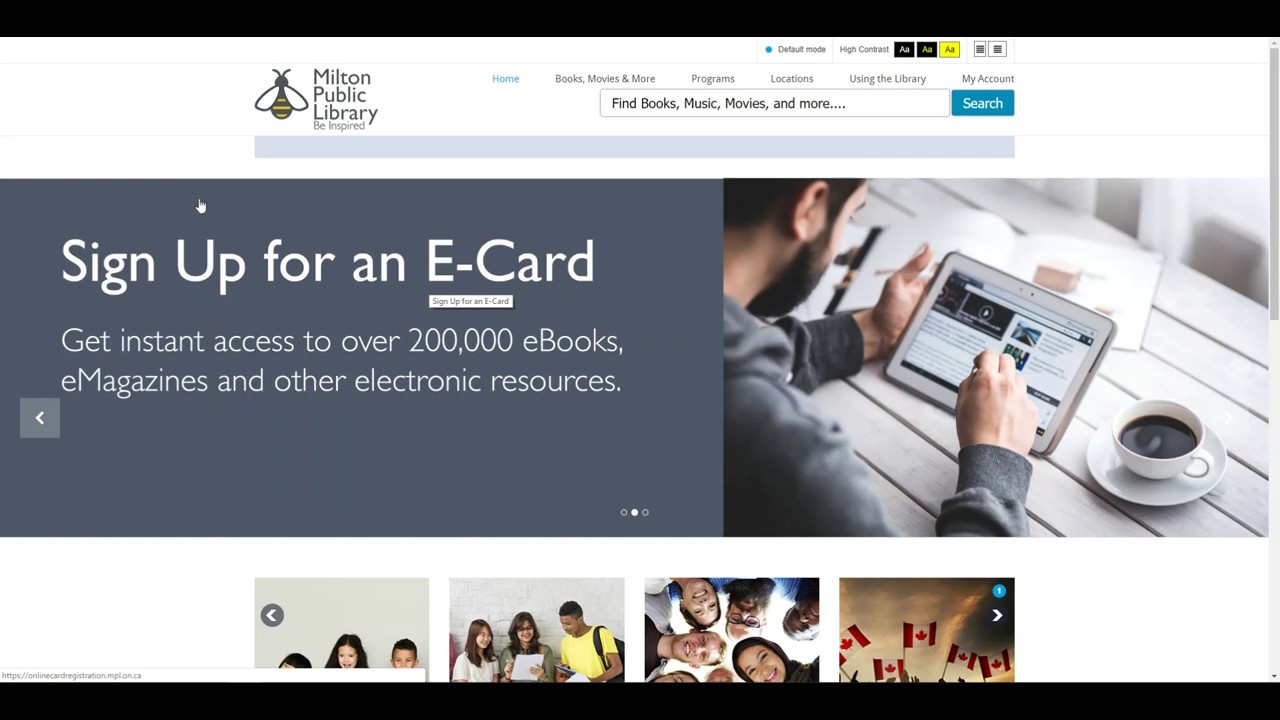"Homepage of Milton Public Library's website, featuring a streamlined design with black banners at the top and bottom extending from left to right. Centered prominently in the upper banner is the text 'Milton Public Library' with the slogan 'Be Inspired' directly underneath. Adjacent to the text is an overhead shot of a bumblebee with distinctive black and yellow stripes, two wings, a round head, and antennae at the top. 

To the right of the library's name and logo is a search bar with placeholder text ‘Find books, music, movies and more,’ and a light blue search button. Above the search bar are navigation links in blue for 'Home', 'Books, Movies, & More', 'Programs', 'Locations', 'Using the Library', and 'My Account'.

The center section of the page features a bold white text against a gray background that reads 'Sign up for an e-card' promoting instant access to over 200,000 eBooks, e-magazines, and other electronic resources. To the right, there is an image of a man using a tablet with a cup of coffee beside him, suggesting a comfortable and modern digital reading experience.

Below this section, there are four smaller images depicting various topics, adding visual interest and inviting further exploration of the library's resources and programs."